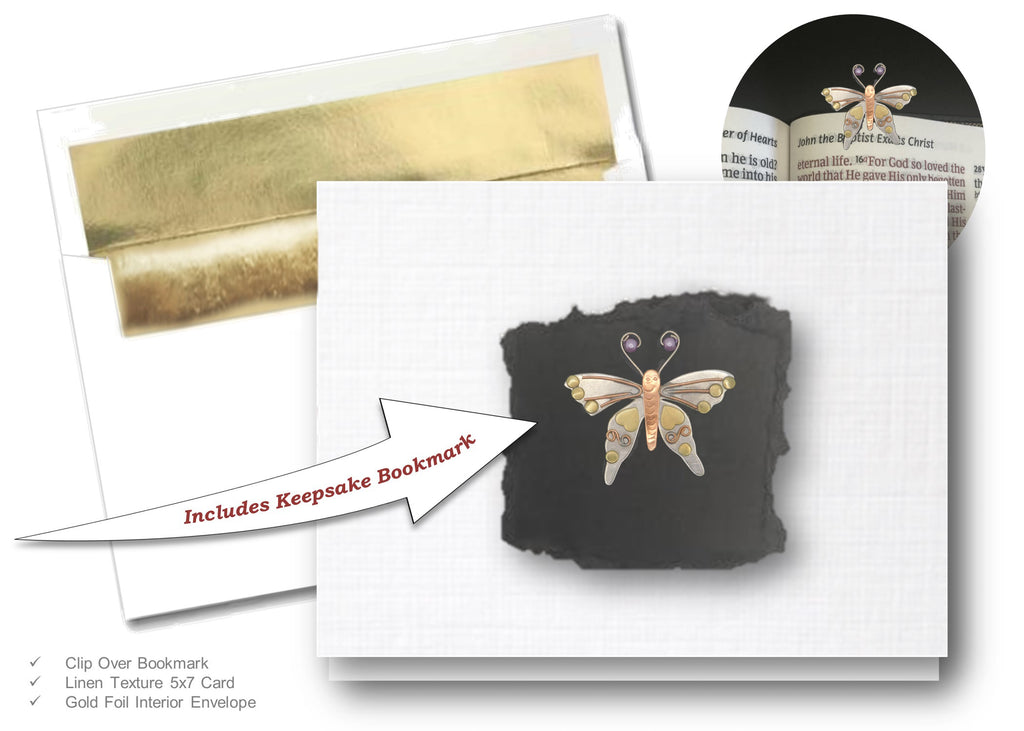This image showcases a detailed greeting card set against a plain white background. Central to the composition is a white 5x7 card featuring a butterfly logo set against a squarish black section. Surrounding the card are various components of the set: 

In the upper right corner, there's a smaller circular image displaying an open Bible with text highlighting "John the Baptist" and "Christ," presumably accompanied by verses, and labeled to include a keepsake clip-over bookmark. This bookmark features a butterfly with heart designs.

In the upper left corner sits the white envelope, distinguished by a gold foil interior and a gold seal. 

Detailed descriptors are located in the lower left, featuring three check marks for the attributes: "clip-over bookmark," "linen texture 5x7 card," and "gold foil interior envelope." 

The entire set appears to be a cohesive invitation or greeting card ensemble with an elegant design focused on the butterfly motif and quality material highlights.